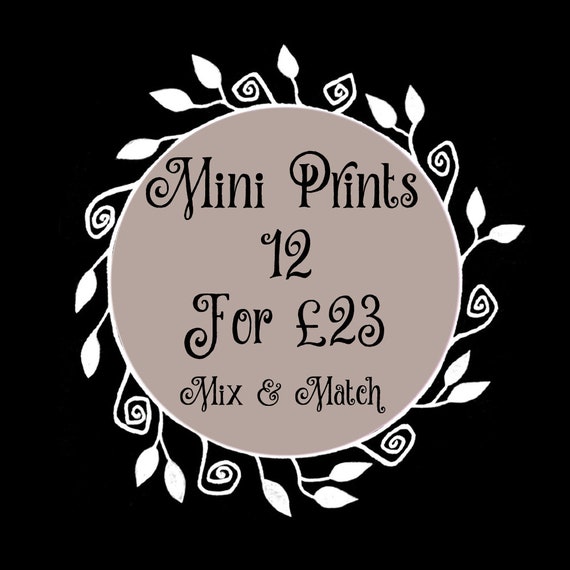The image depicts a store advertisement featuring a sophisticated design. At the center is a large, gray circle containing black text in a highly stylized and flourishing font that reads, "Mini Prints 12 for £23, Mix and Match." The outer edge of this circle is adorned with intricate white designs, including spirals, leaves, and floral motifs, creating a decorative, plant-like border. This detailed circle sits against a stark, solid black background, giving the entire placard a striking and elegant appearance suitable for a high-end store setting.